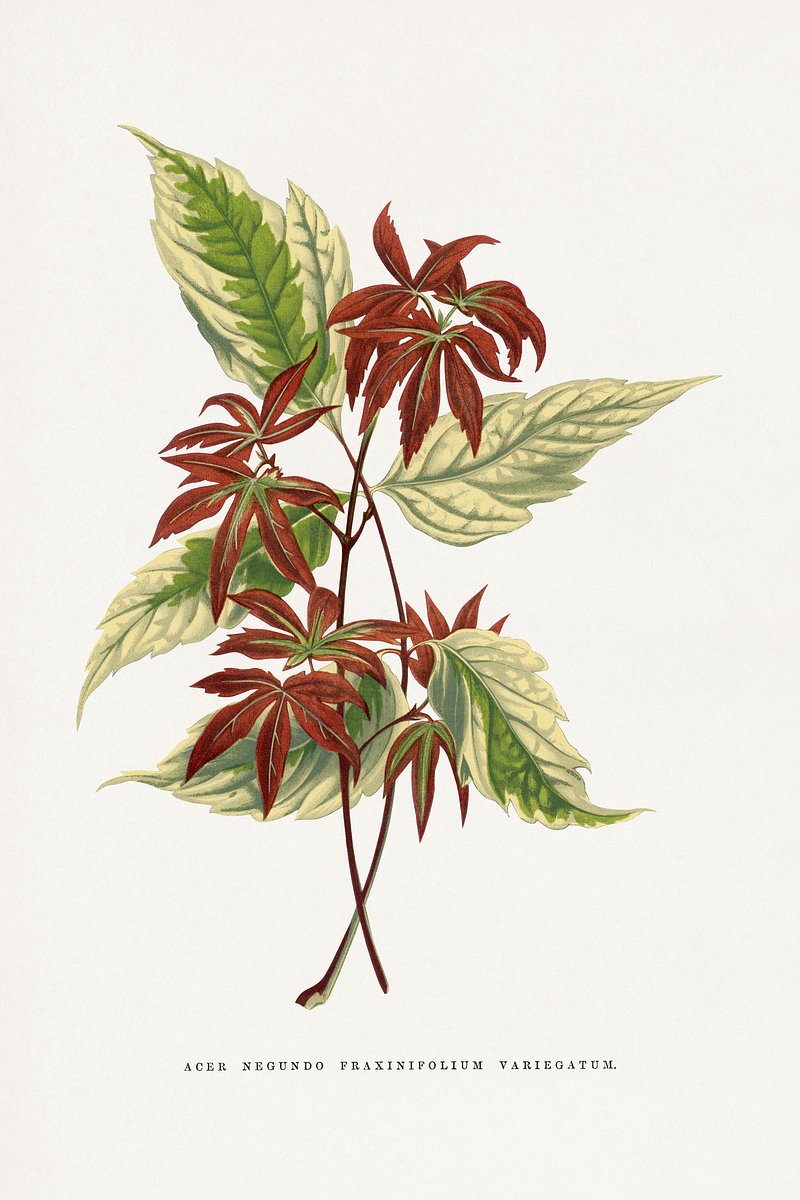This is a detailed painted illustration of a plant specimen on off-white paper. It features two distinct types of leaves, suggesting it could be different species within the same illustration. One set of leaves resembles a maple or marijuana-like formation with an amber color, having a structure with greenish-red stems. These leaves display shades ranging from very light pale yellow to a dark green, and some appear in a very dark maroonish brown hue, indicating variation in leaf age or type. The other type has large, jungle-dense, elephant ear-like leaves in a forest green color, with soft-toothed edges that turn white towards the tips. Both leaf structures are depicted as not being densely packed, each having a notable spread. The background of the image is a dark white or light cream color. Below the intricate foliage illustration, there is scientific text in black capital letters, reading "Acer negundo proxenopoleum variegatum," identifying the plant specimen.